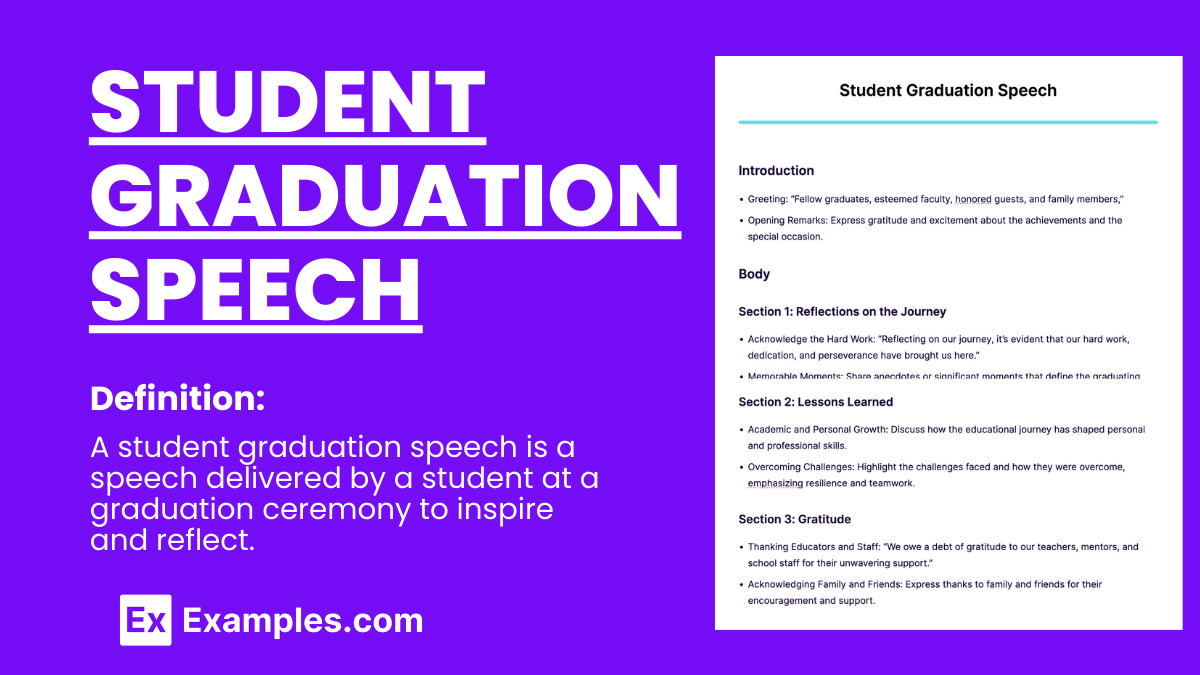The image features a bright bluish-purple background with white lettering, prominently displaying the title "Student Graduation Speech" in large, underlined, all-capital letters on the left side. Below the title is the definition: "A student graduation speech is a speech delivered by a student at a graduation ceremony to inspire and reflect." At the bottom left, the text "examples.com" is displayed. The right side of the image showcases a white document exemplifying a student graduation speech. This document is organized with headings such as "Introduction," which begins with a greeting to graduates, faculty, guests, and family members, and continues with "Body" sections, including "Reflections on the Journey," "Lessons Learned," and "Gratitude." The entire composition features only the colors white, black, and purple, with a turquoise bar symbol at the very top of the image, and no additional text or images.